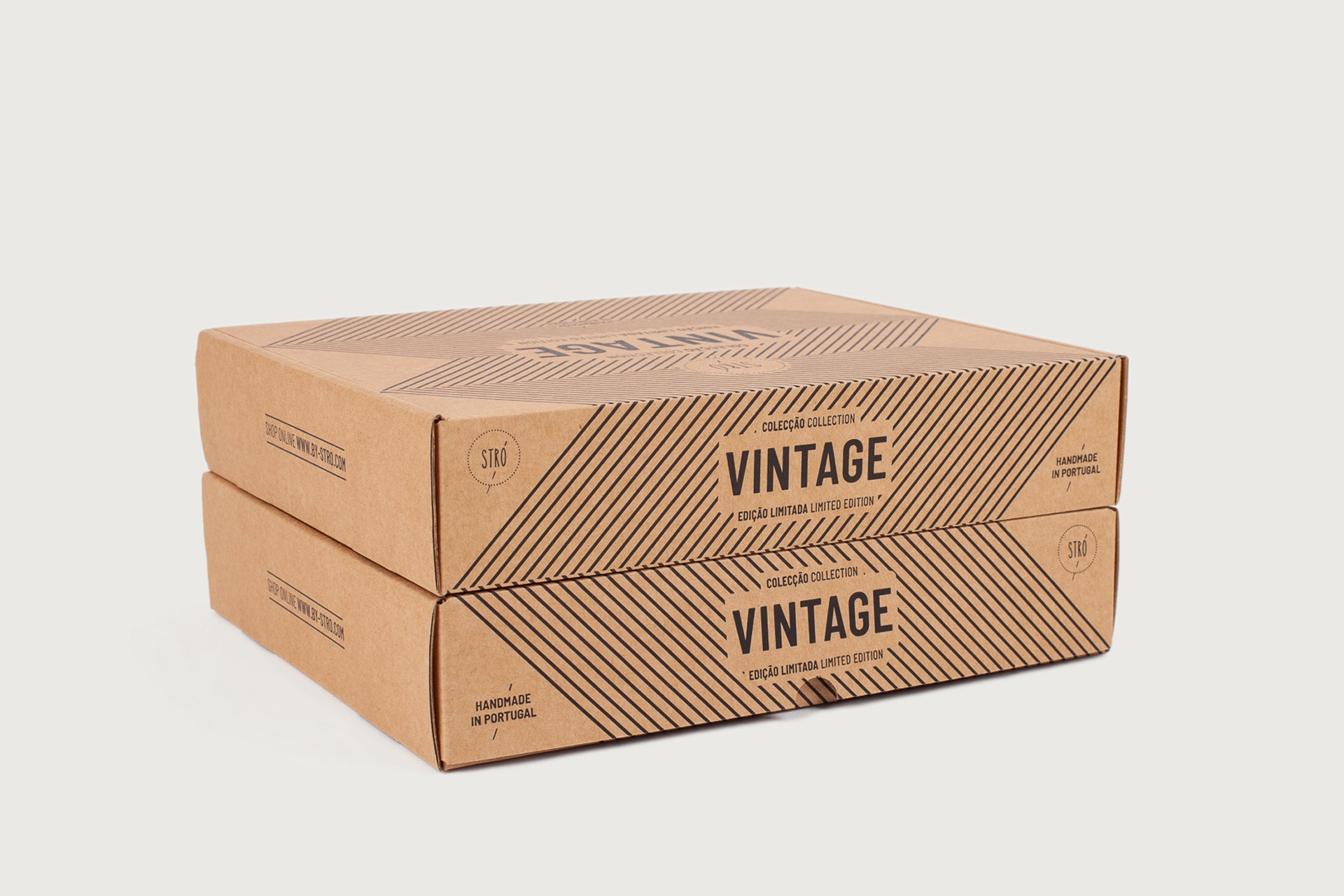The image showcases two stacked boxes, one positioned on top of the other. The photograph is taken from the back side of the boxes, evidenced by the angle that reveals part of the top box's surface and the back-facing label. The topmost box has the word "vintage" printed on its top, oriented towards the upper left side of the image, visible from a slight slant. The word "vintage" also appears upright and prominently on the back side of the top box, which faces the camera directly. Intriguing slanted lines frame the word "vintage," adding a touch of retro design to the boxes. Additionally, a portion of the right side of the top box is visible, featuring more text or details that contribute to the overall aesthetic.